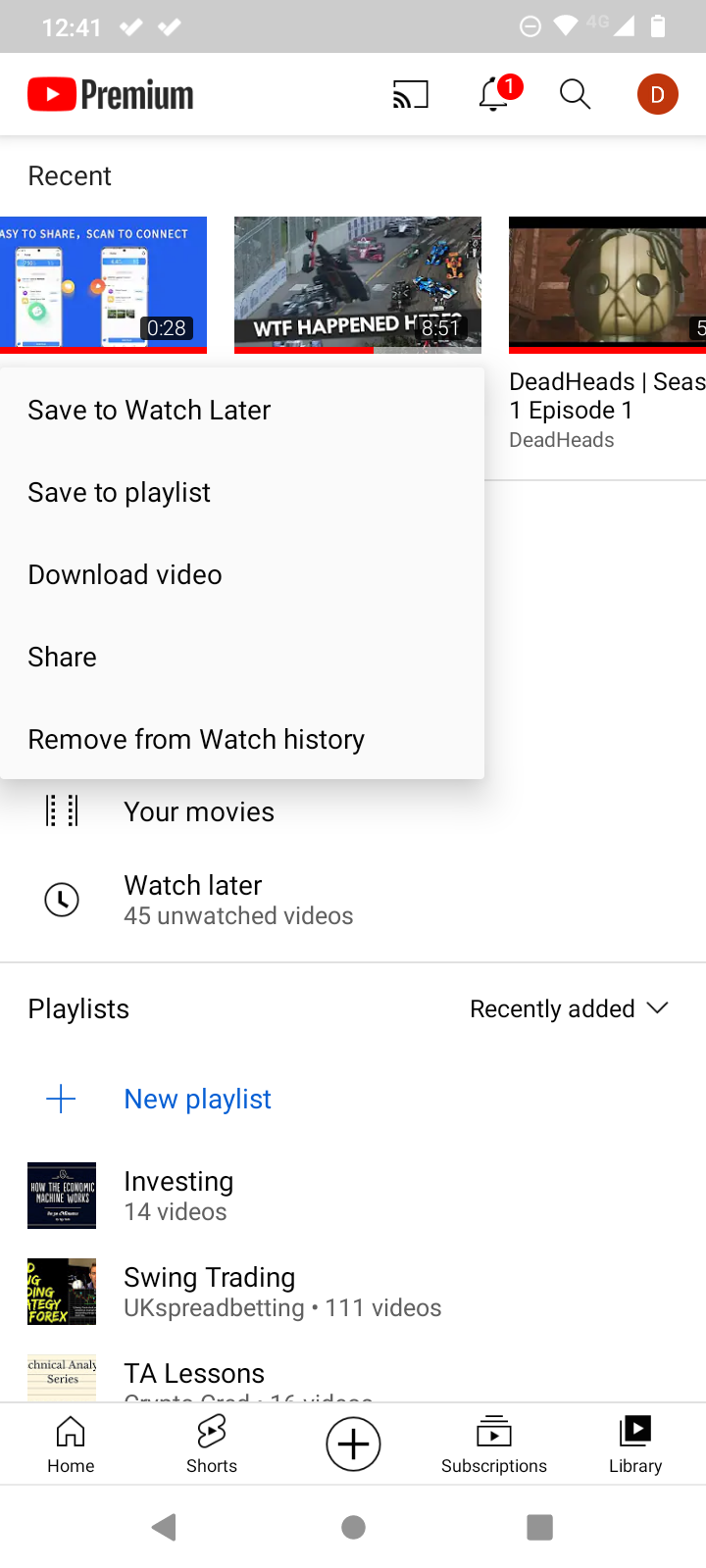This detailed caption describes a screenshot captured from an Android device displaying the YouTube app interface with various metrics and features visible:

---

**Screenshot Description: YouTube Interface on Android Device**

The screenshot showcases a YouTube interface on an Android phone. Detailed elements of the interface are as follows:

- **Top Status Bar**: 
  - On the top left, the time is displayed in white font, reading "12:41", followed by two white check marks on the right.
  - On the top right, there are icons indicating full Wi-Fi signal, full 4G cellular service, and an almost fully charged battery.

- **YouTube App Interface**:
  - Below the status bar on the top left, a white bar indicates YouTube Premium membership, featuring a red Play button and the word "Premium" in black text to its right.
  - Next to this bar, a series of icons are arranged sequentially, including: 
    - A Chromecast button
    - A bell icon with a notification (one)
    - A magnifying glass (search) button
    - A profile picture depicted as a burnt orange circle with a white letter "D" in the center.

- **Recent Activity and Video Options**:
  - Underneath the YouTube Premium bar, the screen shows a list of recently watched videos. The most recent video appears to have been selected, displaying options such as "Save to Watch Later," "Save to Playlist," "Download Video," "Share," and "Remove from Watch History."

- **Additional Library Options**:
  - Below these options, the interface provides access to the user's "Movies" and "Watch Later" sections, with "Watch Later" indicating 45 unwatched videos.
  - Further down is a list of playlists available to the user, such as:
    - An "Investing" playlist containing 14 videos
    - A "Swing Trading" playlist with 111 videos
    - A "TA Lessons" playlist
  - Options to create a new playlist are also present.

- **Bottom Menu Bar**:
  - At the bottom, a white menu bar displays primary navigation options: "Home," "Shorts," "Plus," "Subscriptions," and "Library."
  - Below this menu bar, in light gray, are additional navigation buttons: a left-facing arrow (Back), a circle (Home), and a square (Recent Apps).

---

This caption provides a comprehensive and clear description of the elements visible in the YouTube screenshot on the Android phone.